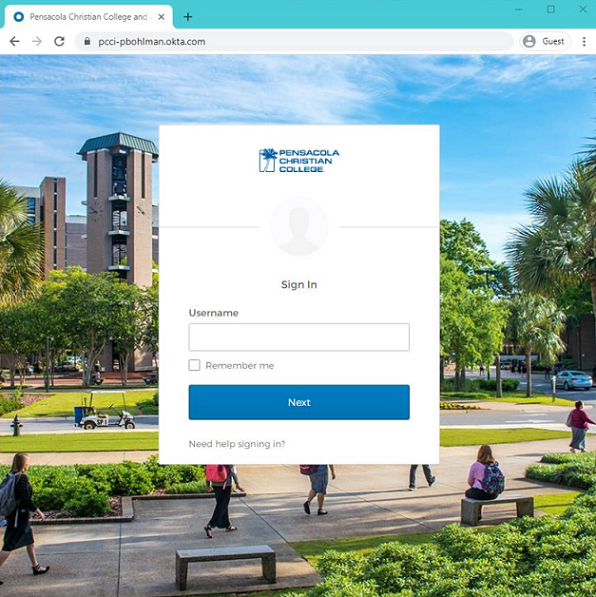The image features a website with a visible search bar containing the text "Pensacola Christian College." The website corresponding to the search is displayed on a white pop-up overlay. At the top of the pop-up is the name "Pensacola Christian College" alongside an image of a palm tree. The pop-up also includes a very faded, generic person icon, which is barely visible due to its whiteness. Flanking this faded icon are two gray lines on either side. Below, the pop-up provides options to "Sign In" with a designated space for entering a username. There is a "Remember Me" checkbox and a blue "Next" button. At the bottom, a link reads "Need help signing in?"

This pop-up appears over a background photograph of the college campus. Visible in the backdrop are modern, contemporary buildings; one notable structure resembles a tower with a flat roof. The extensive campus grounds show students walking with backpacks and a girl in a pink sweater sitting on a bench. A small roadway is observable with maintenance vehicles, likely golf carts, and several cars driving into the campus. The setting is bathed in sunlight under a clear, blue sky with a few scattered clouds, indicating a bright, pleasant day.